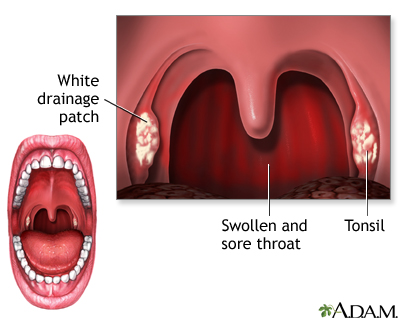The image is a detailed medical diagram of a mouth, divided into two sections. On the left side, there is a smaller depiction of an open mouth where the white teeth, red tongue, and the inner red color of the mouth are visible, along with the lips above and below the teeth. On the right side, there is a larger, close-up illustration of the throat. This part of the diagram marks several key features: a "white drainage patch" on one side, indicated by a line pointing to its location inside the mouth; "swollen and sore throat," highlighted in red with a line pointing towards the throat; and the "tonsil," with a line pointing to its position. There is also text at the bottom right that reads "ADAM" with a small green leaf beside it, indicating the source of the diagram.